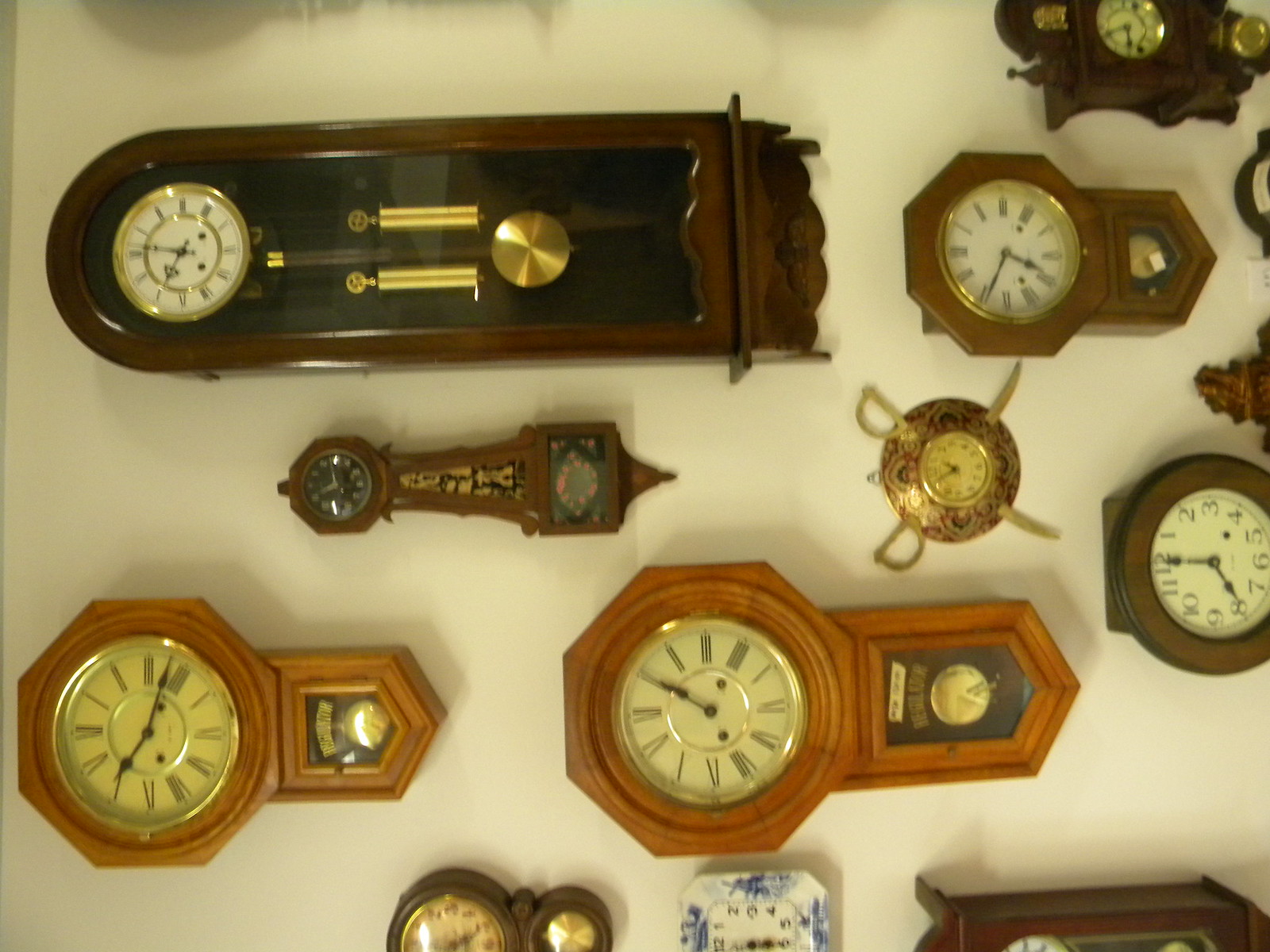This image, taken sideways, showcases a collection of around 11 varied old-fashioned analog clocks on a tan wall. These clocks, appearing somewhat blurry in the low light, mostly have wooden frames, ranging from light-colored pine to polished mahogany, often accentuated with gold borders and pendulums. Among the collection, notable pieces include two octagon-topped wooden clocks that narrow into a point, a large grandfather clock with visible gold pendulums and weights, and a brass clock embedded in a shield-like design with crossed swords. Additionally, there's a distinct blue and white ceramic clock resembling the back of a saucer at the bottom of the image. The image orientation requires viewers to tilt their heads to the left to see the clocks properly, adding a unique perspective to this old clock collection.